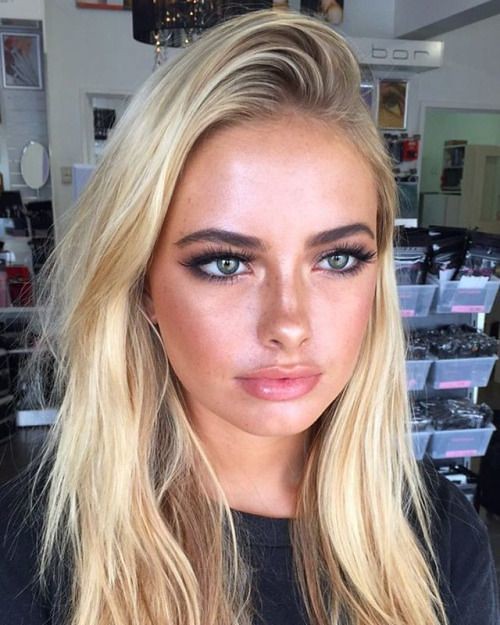In this image, we see a selfie of a young, attractive Caucasian woman with long blonde hair and light green eyes. She is wearing a black shirt and appears to be indoors. Her clear skin and puckered lips are prominently displayed as she gazes into the distance. The image is well-lit, with light reflecting in her eyes, suggesting she might be doing a webcast, potentially a makeup tutorial.

Behind her, there is a shelf filled with transparent plastic totes, some of which have pink labels and appear to contain products, possibly beauty equipment. To the left side of the image, a round mirror is visible, and above it, there is another picture. The setting includes a room with white walls and a doorway leading into an adjacent room with green walls. There is also a sign with the word "BOR" in gray. The overall setting suggests an environment filled with makeup and beauty tools, highlighting the possibility that she might be demonstrating makeup techniques or products.